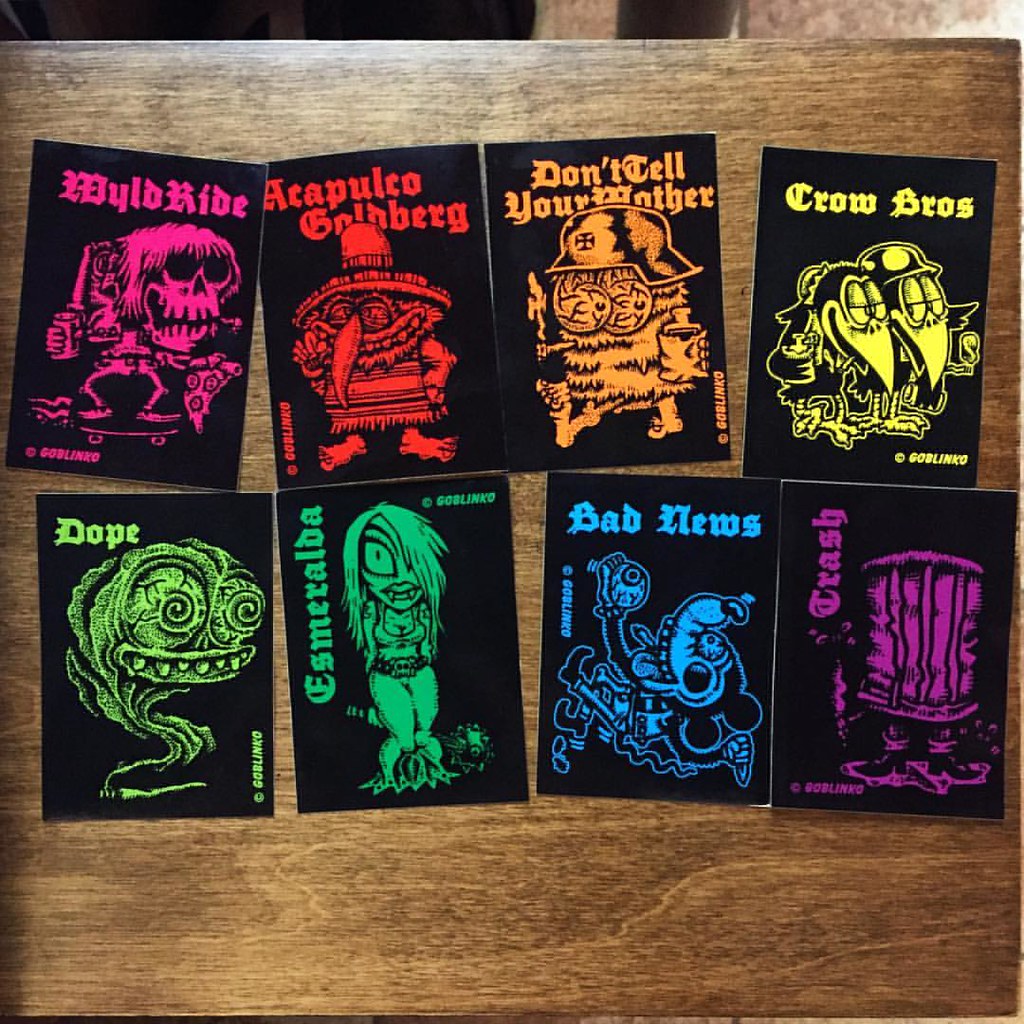This rectangular photograph showcases eight vividly colored trading cards arranged neatly on a medium to dark wood table. Each card sports a black background with fluorescent accents and features unique, cartoonish characters drawn in a horror or scary style. The characters often have exaggerated features like fangs and big eyes, sometimes holding weapons. 

The cards are lined up in two rows of four. In the top row, from left to right:
1. "Wild Ride" – A hot pink card depicting a skeleton on a skateboard holding a beer and a pizza.
2. "Acapulco Goldberg" – An orangey-red card featuring a bird in a Mexican outfit.
3. "Don't Tell Your Mother" – A yellow card showing a Garfield-like cat with a peculiar hat.
4. "Crow Bros" – A yellow-green card with two crows standing side by side.

In the bottom row, from left to right:
1. "Dope" – A bright fluorescent green card portraying a fish-like creature.
2. "Esmeralda" – Another shade of green card featuring a mermaid-like woman with big eyes and long hair.
3. "Bad News" – A bright blue card with an indistinct creature.
4. "Crash" – A purple card displaying a cartoonish trash can with feet.

These intricately designed cards suggest a horror-themed collection, each card vivid and meticulously detailed, contrasting sharply against the dark wooden background.